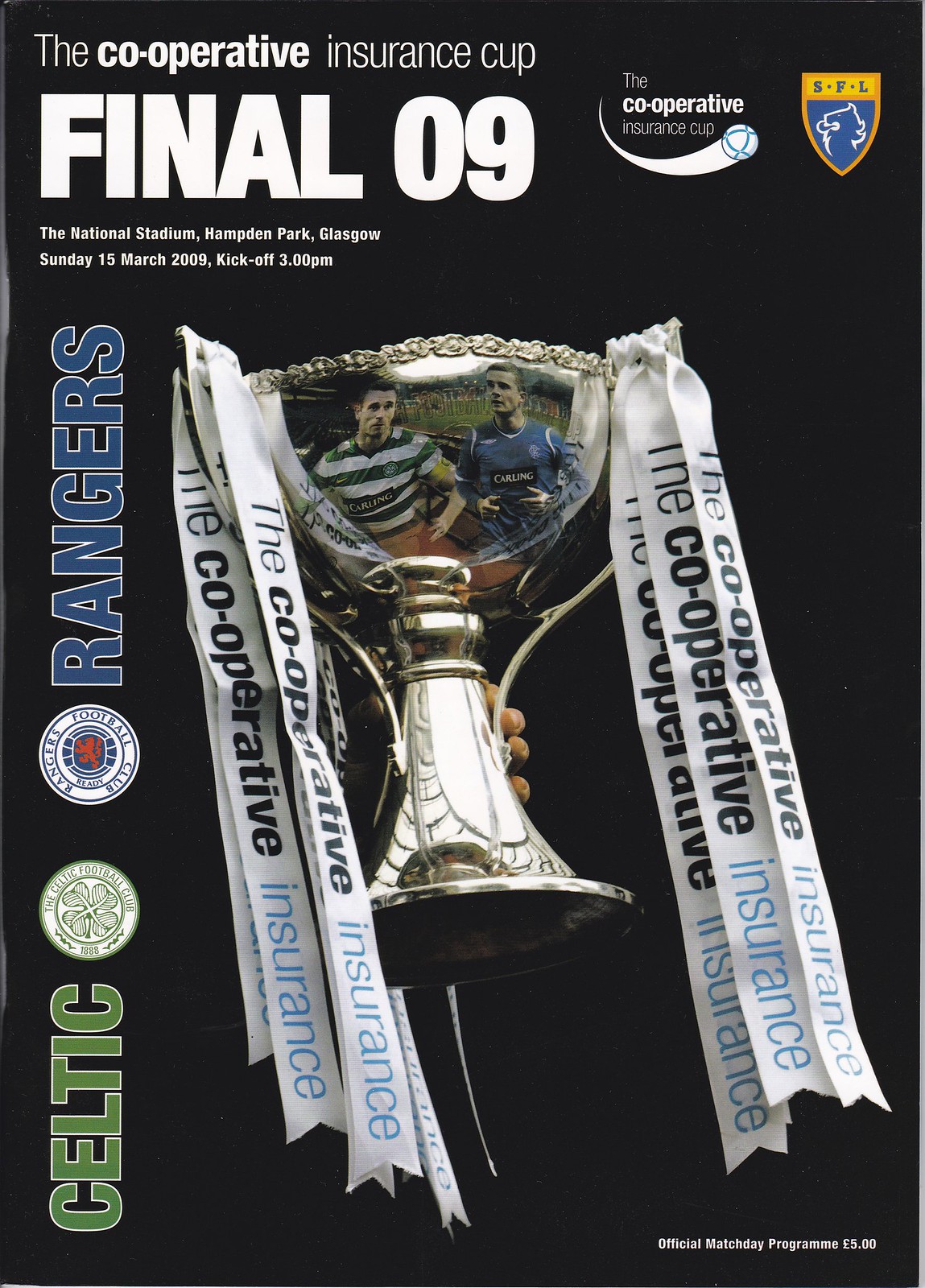The image is a rectangular front cover of an old magazine, predominantly black in color. In the upper left-hand corner, in bold white text, it reads, "The Cooperative Insurance Cup." Below this, in larger white font, it states, "Final 09," followed by smaller text detailing the venue and time: "The National Stadium, Hampden Park, Glasgow, Sunday 15th March 2009, kickoff 3 PM." In the upper right-hand corner, the Cooperative Insurance Cup is mentioned again, accompanied by an illustration of a soccer ball in motion. Adjacent to this is a gold shield with blue text reading "SFL" and an abstract lion's head outline.

Along the lower left margin, the word "Celtic" is printed vertically in green, adjacent to the Celtic Football Club's white circle logo featuring a green four-leaf clover. Above this is the Rangers Football Club’s logo: a white circle with red lions inside a blue soccer ball and the word "Rangers" above it in blue text.

The cover's central image is a gleaming silver cup, reflecting the faces of two Caucasian men. The man on the left wears a green and white horizontally striped shirt with "Carling" printed on it, while the man on the right dons a blue jersey, also bearing the "Carling" logo. White streamers hang from the cup's corners, displaying "the Cooperative Insurance."

In the lower right corner, the text "Official Match Day Programme, £5" is prominently displayed in white.